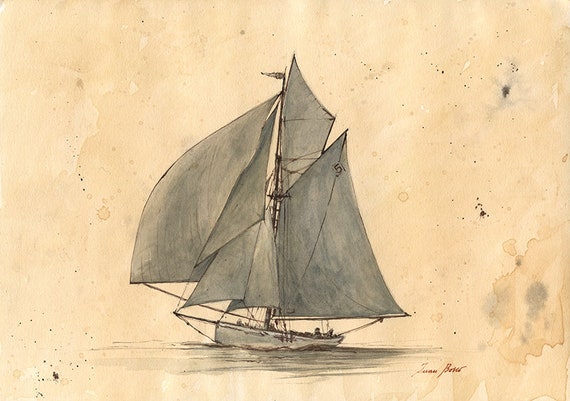This image features a meticulously drawn sailboat rendered on an aged, yellowing sheet of paper adorned with various stains and marks. The sailboat, distinguished by its numerous flags, appears to be floating serenely on still waters. Adding a touch of authenticity and personal connection, a small signature is present in the bottom right corner of the page. The artwork evokes a sense of timeless beauty, capturing the essence of a bygone era with its weathered appearance and intricate details.